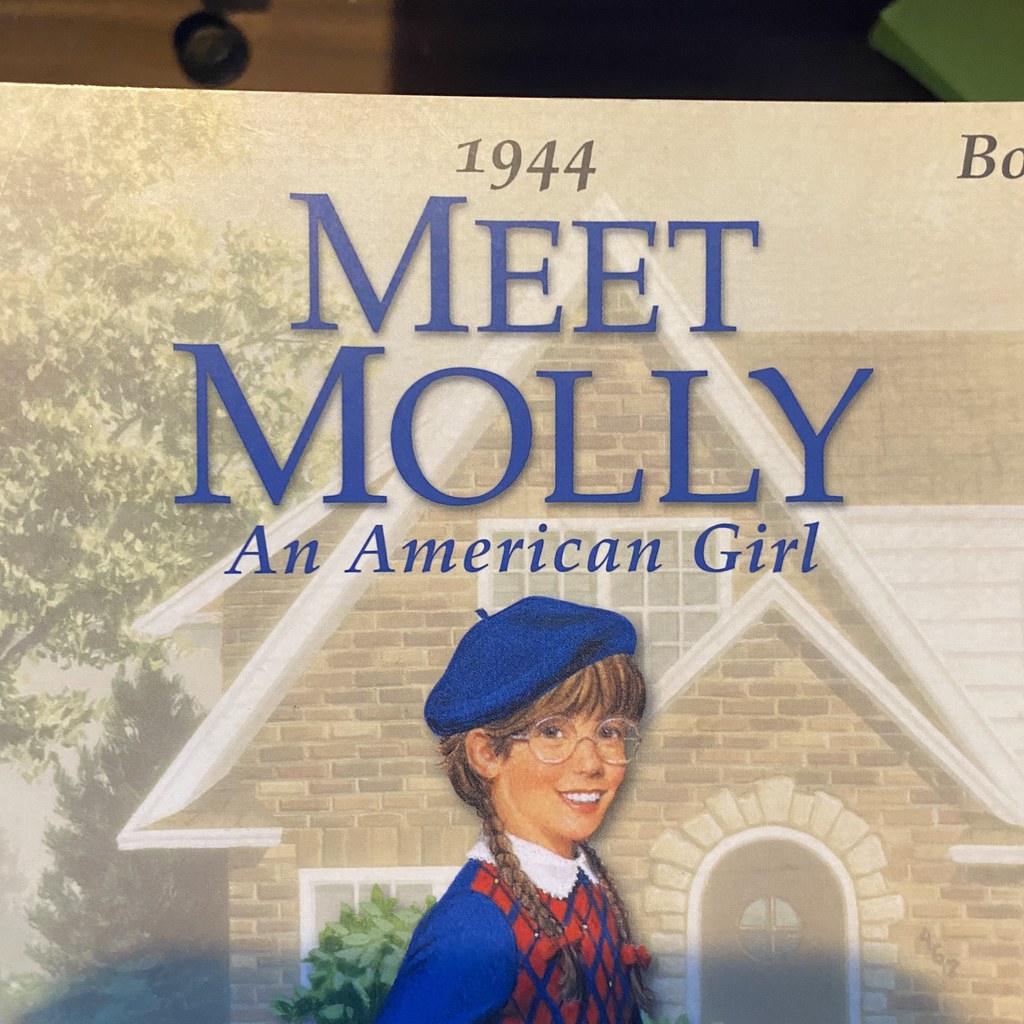This square photograph showcases the cover of an "American Girl" book titled "1944, Meet Molly, An American Girl" in blue text at the top. The central image depicts Molly, a young girl around 10 or 11 years old, standing in front of a brown brick, Tudor-style home with multiple pointed roofs and dark shingles. The house features a dark brown, rounded front door with a circular, cross-framed window, and an adjacent window partially obscured by a shrub. To the left of the house, a large tree with green foliage stands tall. Molly, facing slightly to the right but looking directly at the viewer, sports a blue French beret, round-framed glasses, and her brown hair is styled in pigtailed braids adorned with red ribbons. She is dressed in a white collared shirt beneath a red and blue plaid sweater.